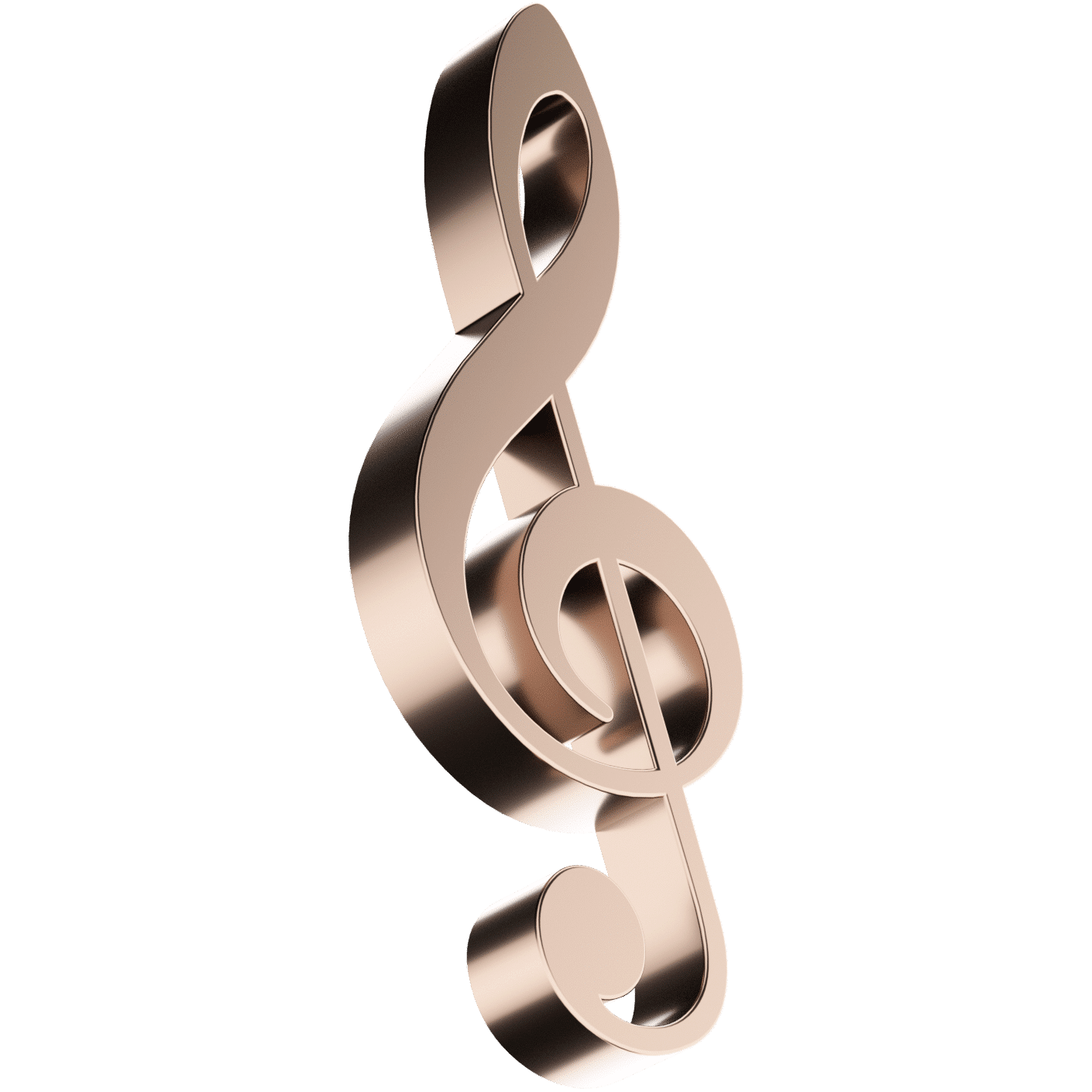The image depicts a large, digitally created treble clef symbol, prominently displayed against a pristine white background. This metallic music symbol is rendered in a captivating blend of rose gold, silver, and copper tones, with a satin-like finish that gives it a smooth, shimmering appearance. The clef is positioned at an angle, leaning towards the bottom right corner of the frame with the top part nearer to the top left, creating a dynamic sense of depth and dimension. The gleaming surface alternates between areas of sheen and shine, enhancing its ornamental quality and lending it a fancy, almost decorative aura. The left side of the treble clef is particularly emphasized, showing thickness and subtle shadowing that highlights its three-dimensional structure. Overall, the clean, shiny look and the striking metallic hues make it a visually appealing and elegant piece, reminiscent of a polished, precious ornament.